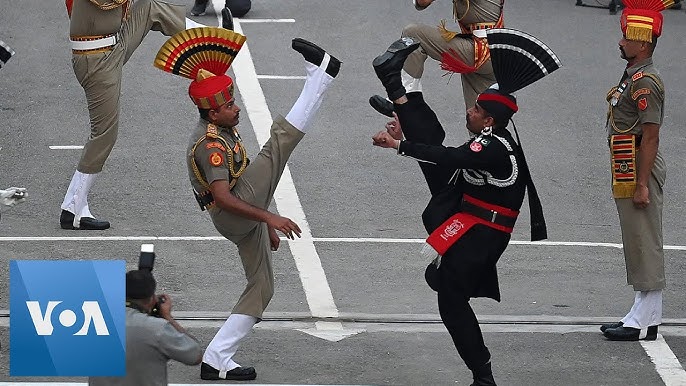The image, which seems to be taken from a clip on a news station possibly labeled VOA, captures a group of men in military garb, likely from a foreign country, performing a high-kicking routine on a street marked with white lines akin to those found in a parking lot. Prominently featured are two men with dark complexions, one dressed entirely in black with a red belt, and the other in light brown, both wearing fan-shaped hats with elaborate designs in shades of gold, black, and red. They are facing each other with their right legs kicked high in the air, displaying impressive flexibility. Both wear black boots. In the background, other men in similar uniforms are also participating in the routine or standing in attention. At the bottom of the image, a man is seen photographing the event.